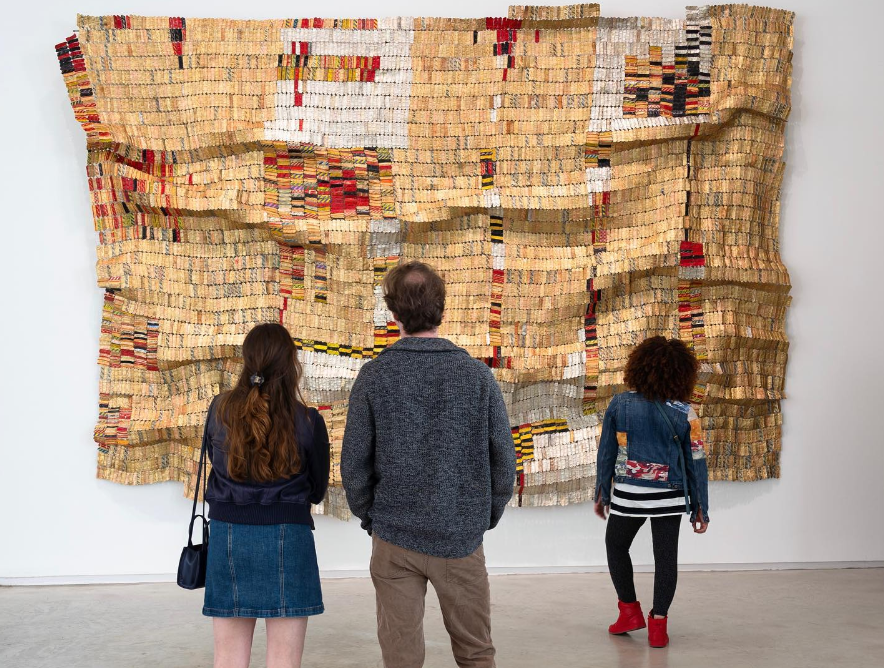In the photograph, three individuals are seen standing in an art gallery, facing a large artwork mounted on a white wall. The focal point of the image is a crinkled, patchwork tapestry composed of numerous small interconnected square pieces in a variety of colors. The tapestry prominently features tan hues, interspersed with white sections and sporadic multicolored patches. On the left side of the image, a woman with long brown hair, dressed in a denim skirt and a black jacket, stands carrying a black purse. Beside her, a man with a gray jacket, khaki pants, and a spot of baldness on his head closely observes the artwork. To their right, slightly separated, stands a younger girl, perhaps a child, dressed in red ankle boots, black leggings, a black and white horizontally striped skirt, and a blue jacket adorned with what appears to be patchwork quilt squares. All three have their backs turned towards the camera, immersed in studying the intriguing quilt-like fabric hanging on the wall.